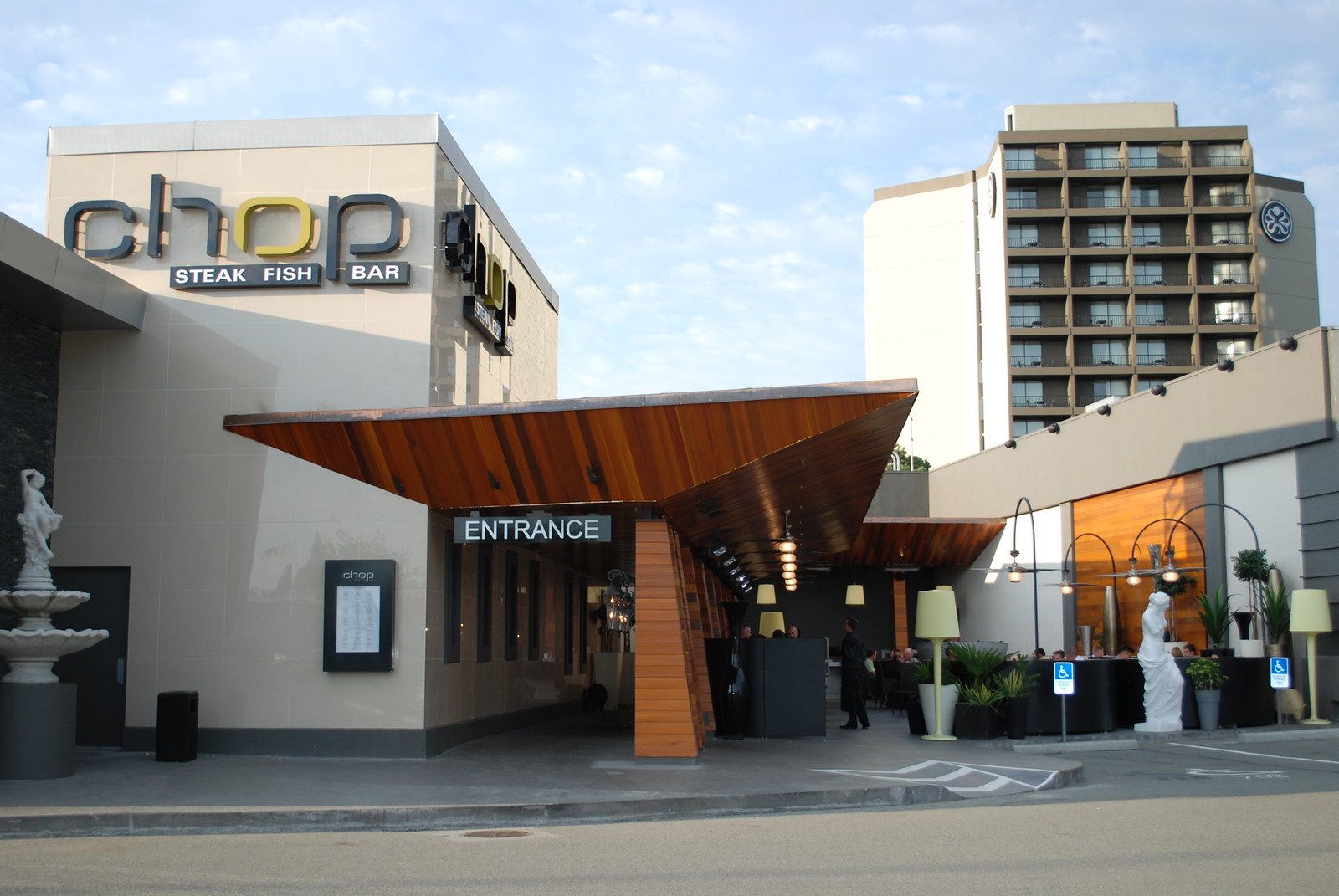The image captures a street view focusing on the front of a modern restaurant called "Chop," with a subtitle "Steakfish and Bar" displayed on a sleek black sign with white letters. The restaurant building features a clean, shiny, and reflective gray exterior adorned with geometric shapes and earth-tone elements. Centrally placed is an ornate wooden entrance with brown pillars and a prominent, black placard overhead that spells out "ENTRANCE" in white text. Unique architectural details include an elaborate wood-trimmed top section above the entrance. To the left of the restaurant's entrance, there is a three-tiered fountain with a seated woman sculpture. Additionally, a statue of Venus de Milo draws attention with its timeless elegance. In the scene, four individuals are gathered outside, seemingly in conversation before entering. To the right of the restaurant, extends a larger building, possibly a hotel, and in the distant background, a taller apartment building with approximately 10 floors is visible, blending into the urban landscape.